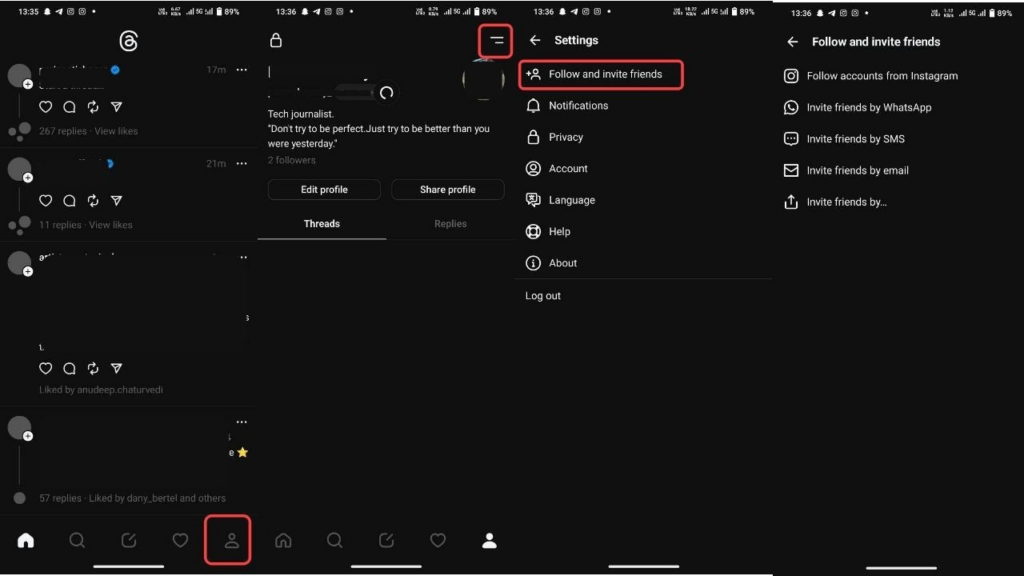This image is a composite of four smartphone screens arranged in a row, each displaying a different step in a tutorial on how to use specific phone functionalities. All four screens share a solid black background, making them appear uniform at first glance. 

The first screen, on the far left, shows a timestamp of 13:35 with several standard smartphone icons on the right, including a battery percentage of 89%. The central icons indicate the phone's status and connectivity. The home button at the bottom left is highlighted in solid white, signifying it is currently selected. Meanwhile, a person icon on the right side of the bottom row is enclosed in a red box with rounded corners, likely indicating the next step.

The second screen, timestamped 13:36, displays the same battery percentage. The red box has shifted to the person icon, now highlighted, guiding the user to select this option. 

The third screen repeats the previous timestamp but focuses on the next action. The red box has moved to the upper right-hand corner, highlighting two lines.

In the fourth screen, the interface directs the user to the "Follow and Invite Friends" section, as indicated by the red box around this option and by the same phrase appearing in the header. 

Overall, this composite image provides a step-by-step visual guide for navigating certain features within a phone's settings.